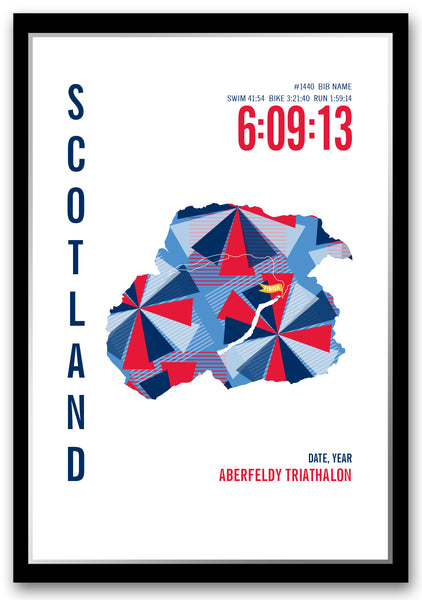This image depicts a framed advertisement for the Aberfeldy Triathlon, featuring a striking and colorful design. The ad is framed in black and set against a white background. On the left-hand side, the word "SCOTLAND" is prominently displayed in capital blue letters running vertically. Central to the design is an arrangement of triangles in shades of red, white, dark blue, and light blue, forming a circular pattern that resembles the tops of beach umbrellas.

In the upper right corner, the advertisement provides race details with the text "#1440 Bib Name" followed by timing splits: "swim 41:54," "bike 3:21:40," and "run 1:59:14." Dominating this section in large red digits is the overall race time: "6:09:13," likely indicating the winning time. The lower right corner of the ad notes the event specifics, with "date, year" and "Aberfeldy Triathlon" highlighted in red text.

This visually engaging poster blends the colors and spirit of the event with essential information for participants and spectators alike.